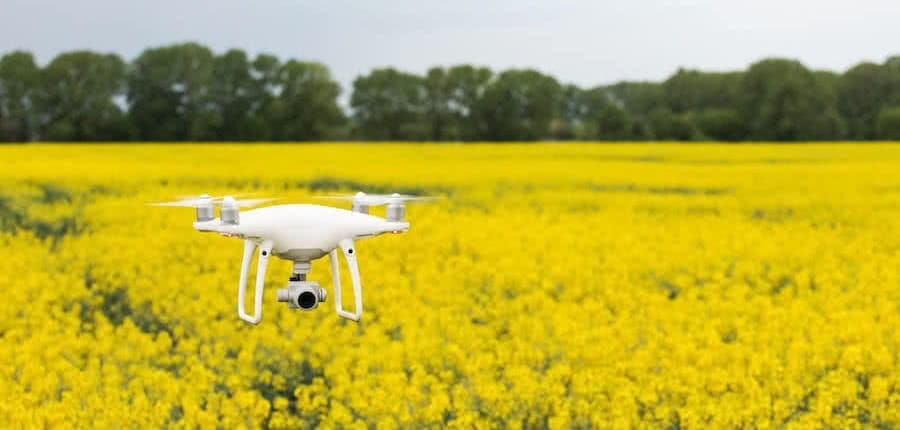The photograph showcases a white drone prominently positioned near the center and foreground of the image, appearing fairly close to the camera. This quadcopter drone features four spinning propellers and two white landing stands, with a camera mounted at the bottom. The camera is distinctly visible with its black lens. The backdrop of the image is a vibrant field, primarily yellow with interspersed patches of dark green grass or foliage poking through, indicating possibly blooming flowers over a grassy bed. About a hundred feet back, a row of dark green trees lines the horizon. The sky above is an overcast light gray, contributing to a diffused lighting effect that slightly softens the scene, although the drone remains sharply in focus.